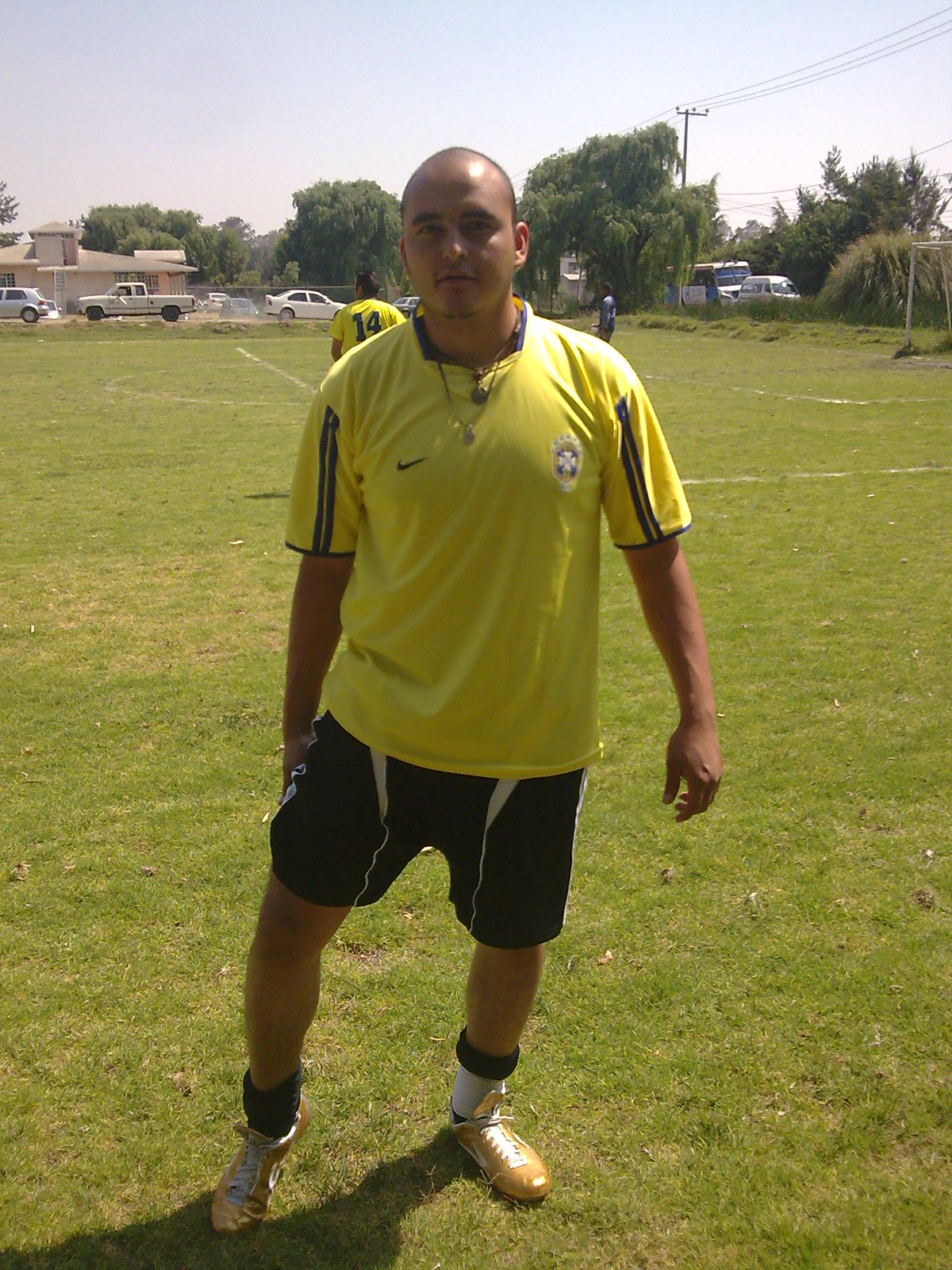The somewhat faded, full-color photograph is taken outdoors during the daytime on a lush green soccer field, under a mostly blue sky with a slight haze. In the background, towards the top of the image, several trees hint at a summertime setting. Various older model vehicles are parked along the field's edges, near a brown building in the far upper left corner. The large open field features a few chalk lines, confirming it as a soccer field, and includes a goalpost on the right side. 

Three men are present, their attire suggesting they are part of the same soccer team. The central figure, and primary focus of the image, is a balding gentleman facing the camera, clean-shaven, and adjusting his right pant leg. He is about 5'8" tall, wearing a yellow jersey with a Nike logo on the right side and a club insignia on the left. His attire also includes black shorts with two white stripes down each leg, black and white socks, and gold shoes. A necklace glistens visibly, accentuated by the sunlight reflecting off his bald spot. 

Behind him, off his left shoulder, is another man in a matching yellow jersey, walking away from the camera with the number 14 visible on the back. Further back, to his right, a man in a much darker, possibly blue or purple, uniform stands closer to the goalpost, though he appears blurry due to the distance. The overall scene captures a moment of preparation or pause on the athletic field, framed by the various elements and characters that add depth and context to the image.